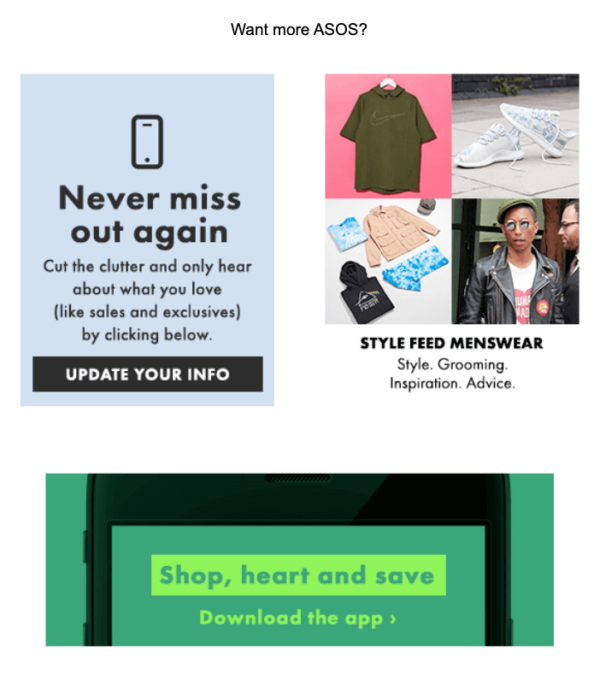This is a high-quality photograph of a section of a website. At the top, the text "Want more ASOS?" is prominently displayed. Below this, there is a blue square featuring the message "Never miss out again" in bold black letters. Within this blue section, there is a graphic of a mobile device, which is shown in a vertical rectangular format. At the bottom of the device graphic, there is a call-to-action button that reads, "Cut the clutter and only hear about what you love, like shoes and exclusives, by clicking below." An adjacent black button says "Update your info."

To the right, the section titled "Style Feed" and "Menswear" is written in a bold black font. Underneath, the subtitle reads "Style rooming inspiration and advice." Below this, there are four photos showcasing different fashion items: a green t-shirt, a pair of white and blue sneakers stacked on top of each other, a wardrobe containing a pair of white and blue pants, a long-sleeve tan shirt, and a black hoodie. Additionally, there is an image of a man wearing aviator sunglasses, a hat, a black motorcycle jacket, and a white graphic t-shirt.

The bottom section of the website encourages shopping and savings with the phrase "Shop hard and save." It also promotes downloading the app, with a green background highlighting the call to action.